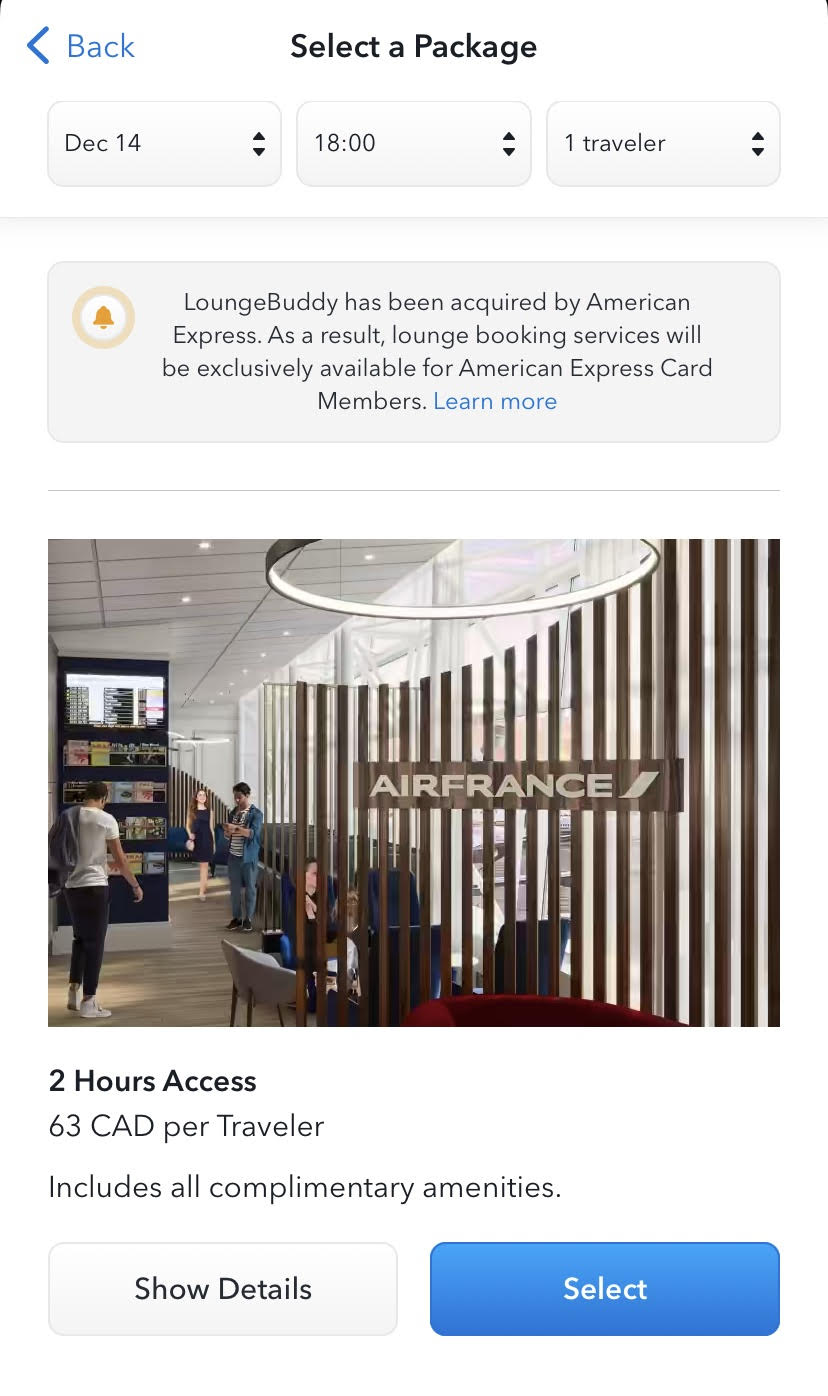The image is titled "Select a Package" and features "Select a Package" in bold, dark black letters. Displayed prominently is the date "December 14th" with a dropdown menu, followed by "1800 hours" and "one traveler," each accompanied by their own dropdown menus.

In the middle of the image, an orange alert bell icon, surrounded by an orange circle, captures attention. Adjacent to it, text in black reads, “LoungeBuddy has been acquired by American Express. As a result, lounge booking services will be exclusively available for American Express card members.” A blue “Learn more” link is positioned below this announcement.

Further down, there is an image of an Air France lounge. The lounge showcases a cozy scene with people relaxing at a small table beside a prominent red couch. The Air France sign is mounted in front of a stylish, wooden privacy screen with visible gaps, providing a modern aesthetic. A large overhead light illuminates the space, complemented by smaller recessed lighting. The scene includes people walking and a substantial shelf, possibly displaying candy or other items.

Underneath the lounge image, details about the service are provided: "Two hours access. 63 CAD per traveler. Includes all complimentary amenities." Two interactive buttons appear below this information: a white box labeled "Show details" and a blue box labeled "Select."